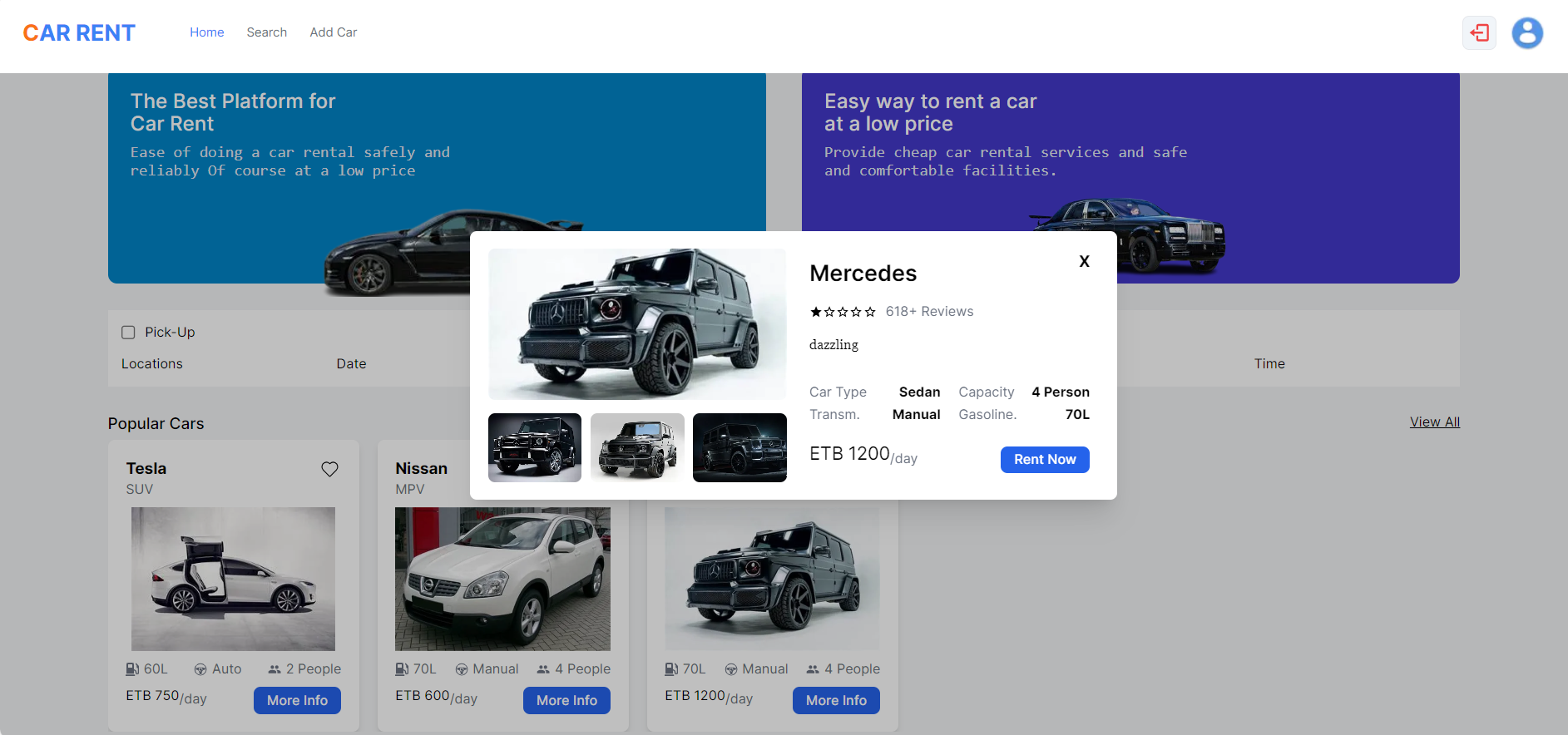**Caption:**

A detailed screenshot of the CarRent website showcasing a variety of elements on its interface. The website's name is displayed at the top left, with "Car" in orange and "Rent" in blue. The navigation bar features "Home" in blue lettering, followed by "Search" and "Add Car" in black. Situated at the far right are a red back button and a profile icon.

The main page prominently features a blue box with white text proclaiming, "Best platform to rent a car, ease of renting a car safely and reliably, of course, at a low price," styled in a font reminiscent of the Commodore 64.

Adjacent is a purple box with white text that markets, "Easy way to rent a car at a low price for a cheap rental car, car rental services, and safe and comfortable facilities."

In the center of the page, a white box overlies the others, displaying a single star rating with 618 reviews, suggesting a lack of customer satisfaction. This box focuses on a Mercedes that is mislabeled as a sedan when it's visibly a Jeep. It specifies the vehicle has a capacity for four persons, a manual transmission, and a 70-liter gasoline tank, priced at $1,200 per day, along with a "Rent Now" button.

The website also highlights popular cars such as a Tesla, Nissan, and the mislabeled Jeep with individual blue boxes containing white lettering for each vehicle's details, including transmission type and fuel capacity, and a "More Info" link.

Overall, the website emphasizes the convenience and affordability of their car rental services amidst some glaring inaccuracies.